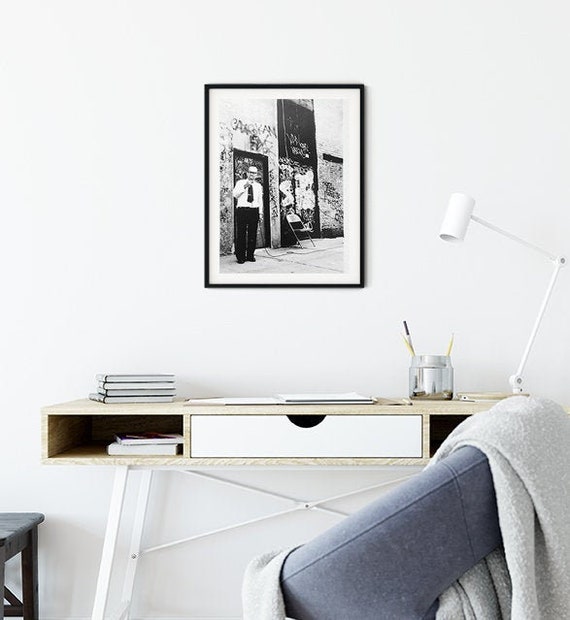This black and white photograph features a minimalist modernist study desk backed against a gray wall. The desk, a tan plywood construction, stands sturdily on a white metal framework with cross paneling. It includes a pull-out shelf in the center and cubby holes on either side for storage. On the desk's surface, an open notebook is flanked by a stack of three thin books on the left and a glass jar holding pens and pencils on the right. Mounted at the top right of the desk is a sleek, white, folding desk lamp poised to provide overhead lighting. In front of the desk, there's a unique pale blue upholstered conical chair, accented by a white blanket draped over it, while just to the left, you can barely glimpse a black wooden stool. Hanging on the wall above the desk is a black and white photograph, framed in a thin black border, depicting a man standing in a doorway along a sidewalk, hinting at a nostalgic scene possibly from the 1920s.